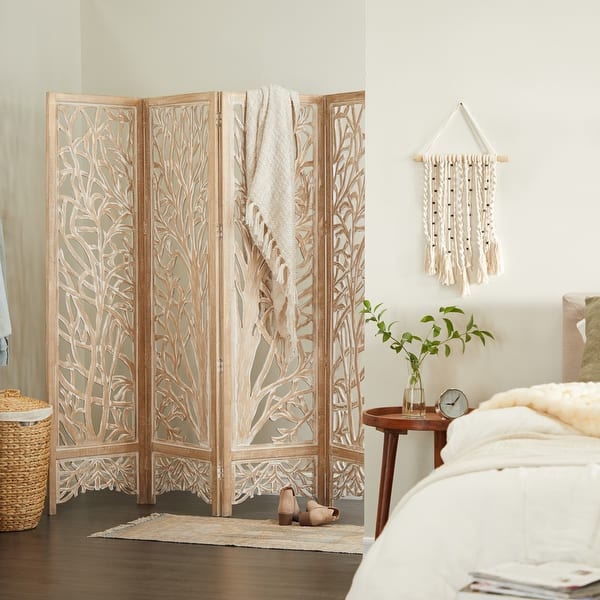This color photograph depicts an airy and light bedroom decorated in monotone colors, primarily ivory and white. The focus is on a four-panel Japanese privacy screen in the back left corner, adorned with a pattern resembling tree limbs. Draped over the screen is an ivory-colored lap blanket with fringes, matching the wall color, bedspread, and a macrame wall hanging. To the left of the room divider is a wicker laundry basket with a lid. In front of the screen, on the hardwood floor, lies a pair of women's shoes and a rug. To the right of this setup is the bed with a tan bed frame, partially visible with its white bedspread. Adjacent to the bed is a tan nightstand, upon which sits a clock displaying "9:05" and a clear vase with a few sprigs of greenery. The room exudes a bright and serene ambiance, complemented by additional details like a potential book or magazine resting on the bed and a subtly visible dream catcher on the wall.